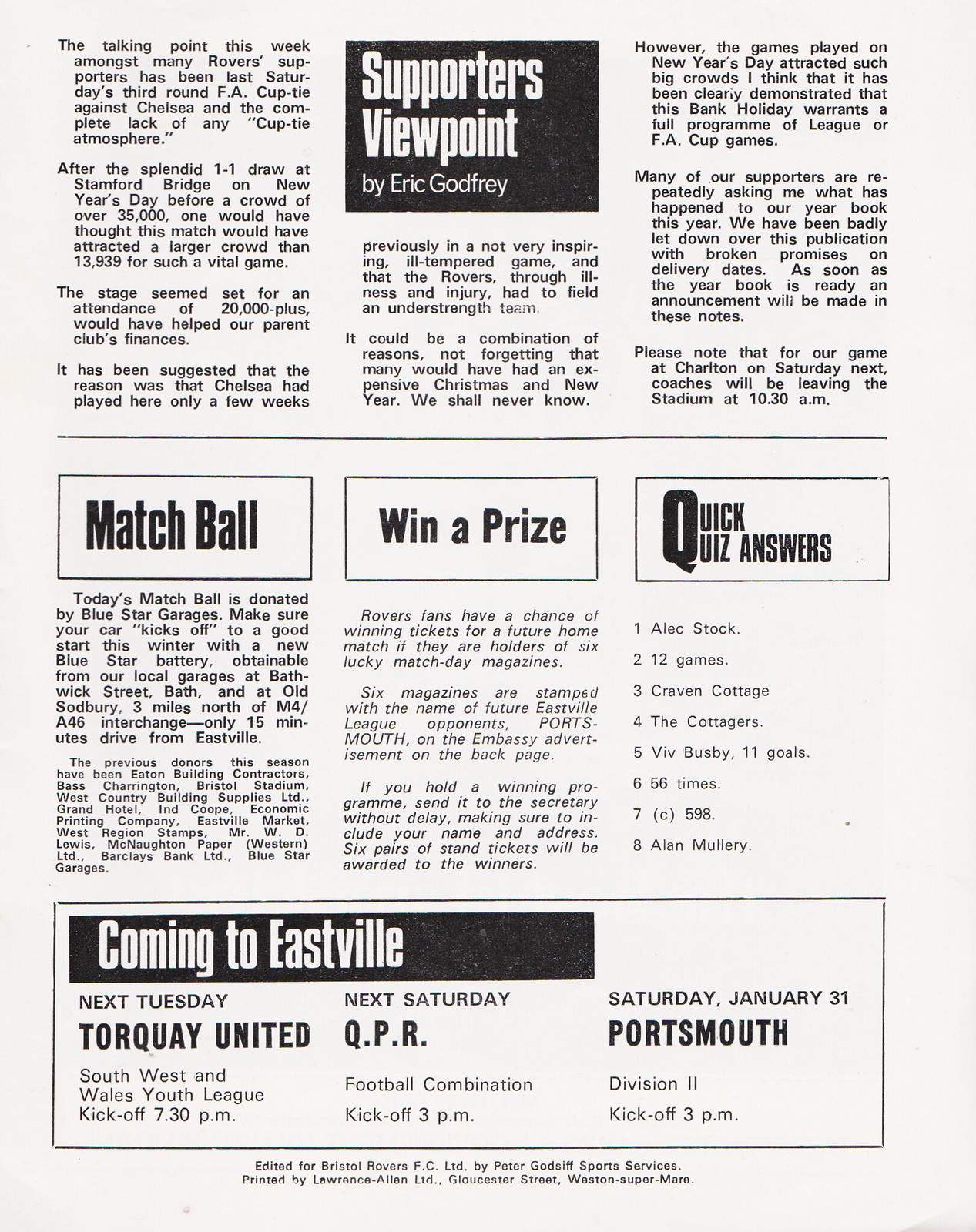The image depicts a page from an old British football magazine printed in black type on a white or off-white background. At the top center, a black rectangular text box with white letters reads "Supporters Viewpoint by Eric Godfrey." This section is flanked by three columns of text. Below this, a thin horizontal line separates the upper section from the lower part. The lower section features three white rectangular text boxes with black lettering, titled from left to right: "Match Ball," "Win a Prize," and "Quick Quiz Answers," each followed by additional text. At the bottom of the page, another black rectangular text box announces upcoming matches: "Coming to Eastville next Tuesday: Torquay United; next Saturday: QPR; Saturday, January 30th: Portsmouth," with further details about the games. The entire layout is reminiscent of a traditional print publication, likely a newspaper or a magazine.